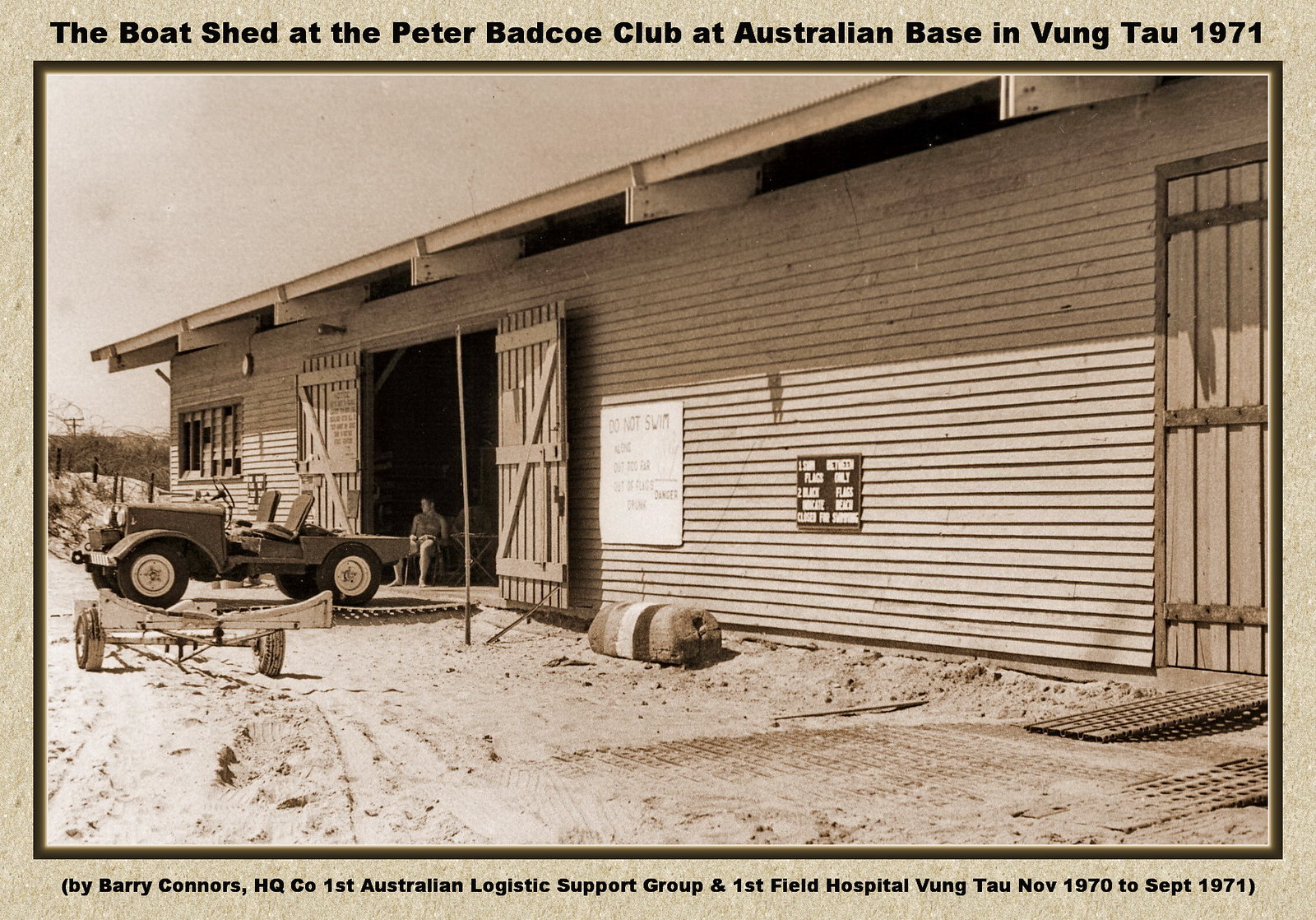The image is a black-and-white photo, with a sepia tint, from 1971. It captures a vintage scene at the boat shed of the Peter Badko Club, located at the Australian base in Vung Tau. The top of the picture is labeled "the boat shed at the Peter Badko Club at Australian base in Vung Tau 1971," while the bottom reads "by Barry Connors, HQ CO, 1st Australian Logistics Support Group and 1st Field Hospital, Vung Tau, November 1970 to September 1971." 

In the foreground, a man in shorts is sitting inside the open shed, relaxing and gazing outside. The doors of the boat shed are wide open, revealing the interior where he is seated. Outside on the left side of the image, a jeep-like vehicle with two seats is parked, alongside a small trailer with two tires. The backdrop shows a dirt ground with sparse dry brush and a few fence posts, suggesting a rugged, perhaps arid environment. Additionally, there is a "do not swim" sign on the shed wall.

This evocative photograph, with its detailed and historically annotated caption, provides a glimpse into the day-to-day life at the Australian military base during the Vietnam War era.